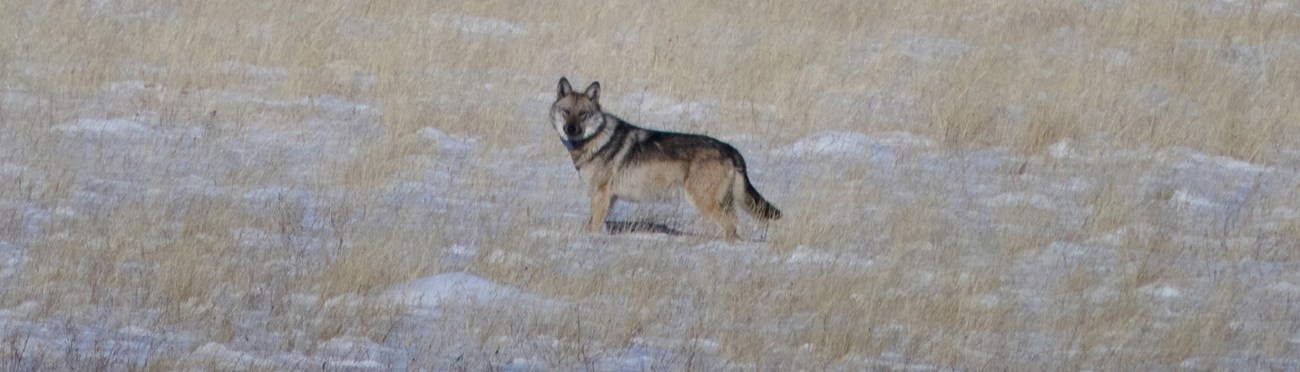This captivating photograph features a lone wolf standing in a wintery field where patches of snow mingle with tall, dead, tan grass. The wolf, with its body angled to the left, faces the camera directly, capturing the viewer with its piercing gaze. Its fur is a stunning mix of black, brown, white, and tan, with distinctive German Shepherd-like markings—a black "saddle" running from the top of its ears down its back to the tip of its tail, and a sandy brown belly extending down its legs. The wolf appears regal and alert, its squinted eyes suggesting the cold air, and its fluffy coat indicating it still carries its winter fur. Though the field stretches beyond the frame, no other wildlife is visible, making the wolf the undeniable focal point against the serene, snowy backdrop.